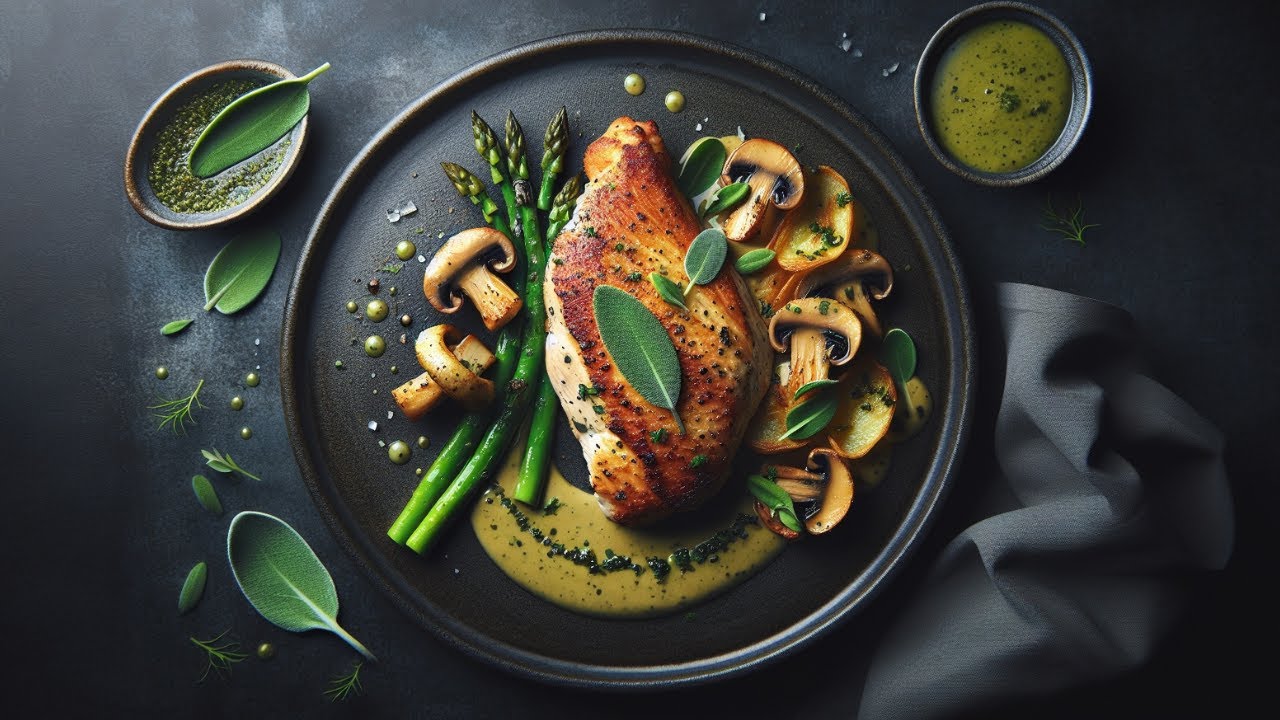The image features a sophisticated overhead view of an exquisite plated dish set against a dark, black-to-gray surface. Central to the visual is a large, black-rimmed plate showcasing a meticulously arranged piece of cooked meat, likely chicken. The meat is accompanied by artfully placed sprigs of asparagus and sautéed mushroom slices, all enhanced by a creamy sauce elegantly drizzled at the bottom. The composition further includes two bowls positioned diagonally from each other; the one on the top right is a black bowl containing a light green liquid flecked with black chunks, while the top left is a reddish clay ramekin holding green seeds. Enhancing its aesthetic appeal, green leaves are scattered on the table to the left of the plate, and a light gray crumpled cloth napkin lies to the bottom right. The entire setting exudes a refined, gourmet presentation.